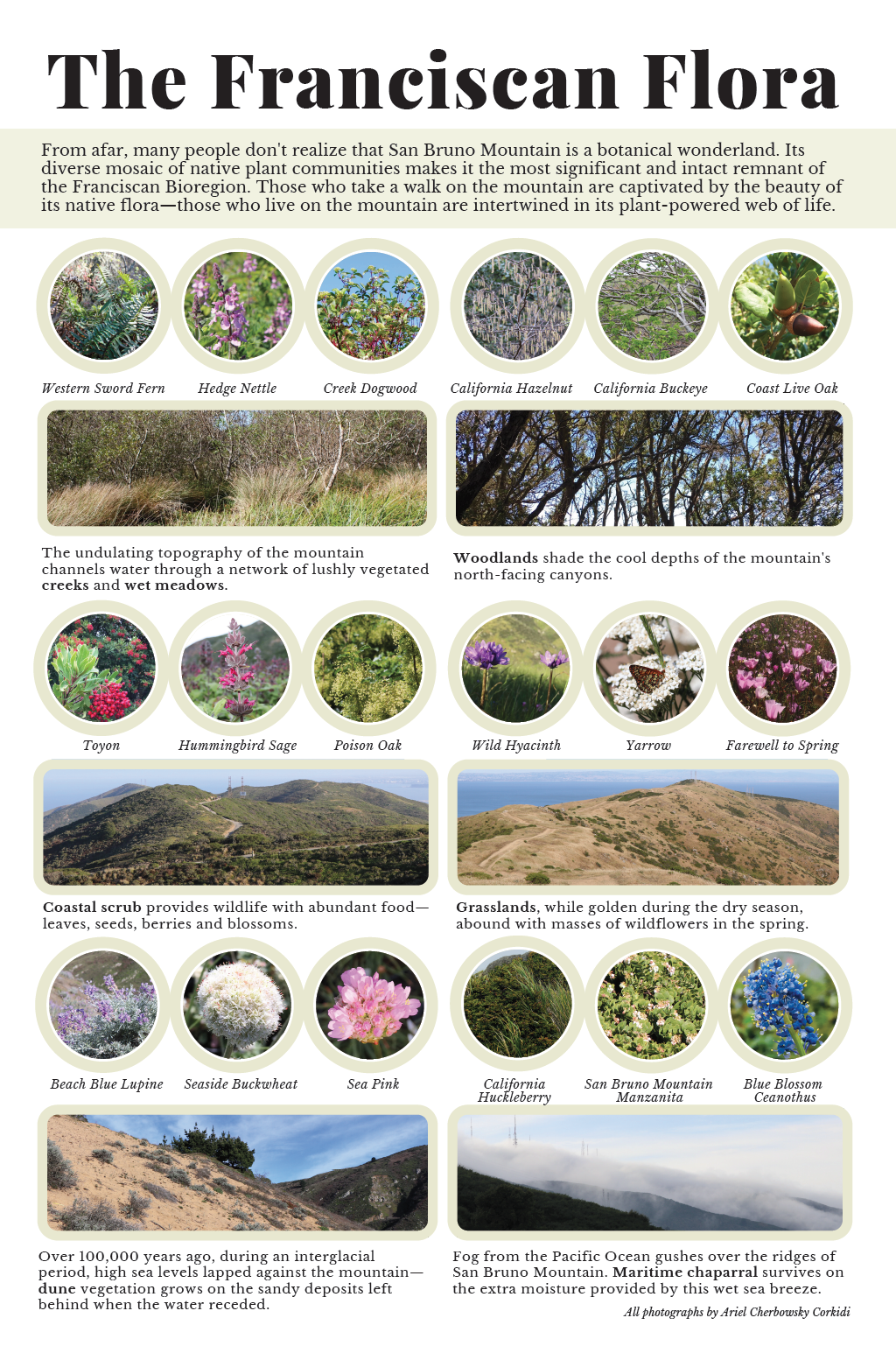The detailed image titled 'The Franciscan Flora' presents a comprehensive outline of the diverse native plant communities on San Bruno Mountain. This mountain, characterized as a botanical wonderland, features a vibrant mosaic of native flora, making it the most significant and intact remnant of the Franciscan bioregion. The introductory text highlights that many people may not initially realize the rich botanical diversity of San Bruno Mountain. It notes that those who walk on the mountain are captivated by its native flora, and the residents live in harmony with its plant-powered web of life.

The image features a detailed presentation of various plants organized into distinct regions and types. Against a white background, there are six circular images bordered in light brown tan, showcasing plants such as western sword fern, hedge nettle, creek dogwood, California hazelnut, California buckeye, and coast live oak. Furthermore, it includes two rectangular photos; one highlighting the undulating topography that channels water through a network of lushly vegetative creeks and wet meadows, and another depicting the shaded woodlands and the cool depths of north-facing canyons.

Additional sections of the image present another set of six plants and two more habitats, followed by yet another set of six plants and two habitats, each accompanied by descriptions. The flora is vibrant, displaying a spectrum of colors including red, lilac purple, pink, blue, and white. These sections cover plants from various terrains — woodlands, coastal scrub, and grasslands. Examples of noted plants include the purple hedge nettle, hummingbird sage, poison oak, wild hyacinth, yarrow, beach blue lupine, seaside buckwheat, and more. These regions together illustrate the overall dry yet flower-friendly terrain of San Bruno Mountain, truly embodying its nickname as a botanical wonderland.